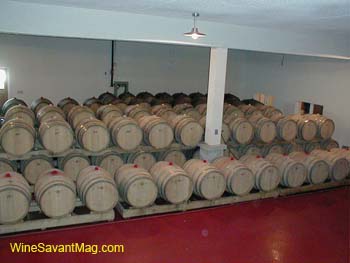The image showcases a utilitarian warehouse room with a stark red floor and white walls, ceiling, and a central column. The room is dominated by stacked wine casks, organized in multiple rows, both vertically and horizontally. The front row of barrels features red corks, while those in the back appear to have white corks. The bottom left corner of the picture contains the text "winesavantmag.com," indicating the possible source of the image. To the left, there's a door with light filtering through its window, while two sets of windows on the right side of the room provide additional illumination. A ceiling light hangs overhead, and at the back, a circuit panel or fuse box with conduit is visible. The barrels are primarily positioned on a wooden platform, and the sheer number of them suggests there are likely more than 100 casks in the room, though it's difficult to count precisely.